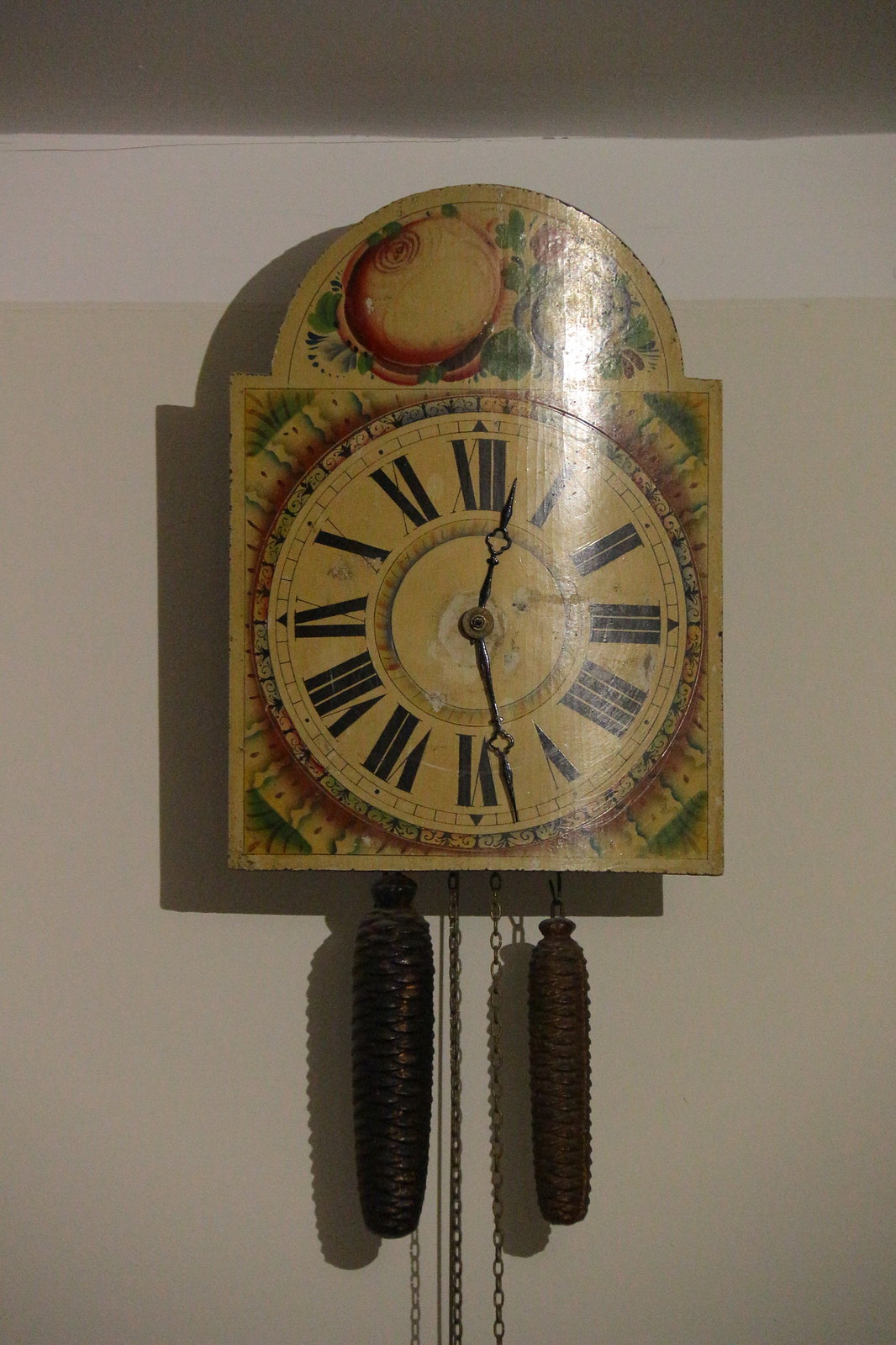The image features an intricately designed analog clock hanging on a beige wall. The clock has a unique and somewhat vintage appearance, with a shape reminiscent of a tote bag. The clock's handle is made of metal and adorned with decorative elements, including fruit and leaves. The main body of the clock is square, while the actual clock face is circular with large black Roman numerals. The time displayed on the clock is approximately 12:29. Below the clock, there are two small, brown decorative pieces hanging from a chain, further enhancing its artistic and antique charm.